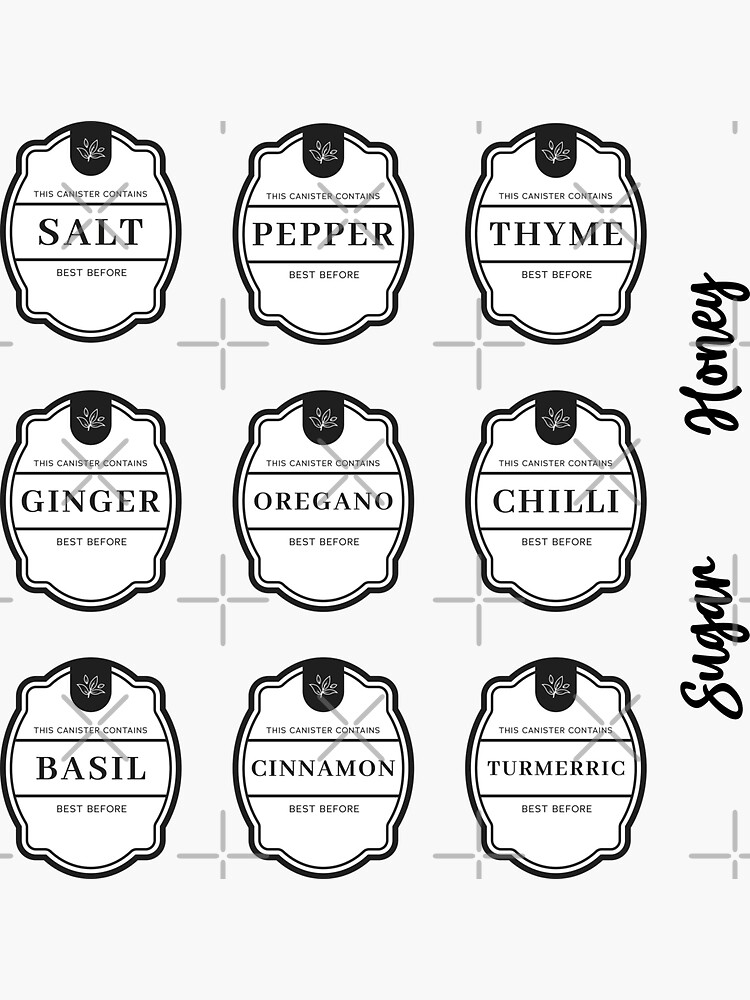This detailed black-and-white image showcases nine distinct labels designed for spice containers, arranged in three rows and three columns, each framed by a simple oval outline with a small shield featuring a leaf at the top. The labels, meant to be printed and affixed to canisters, prominently display the name of each spice in bold text along with a "best before" notation underneath. The spices represented are:

- Top row: Salt (left), Pepper (center), Thyme (right)
- Middle row: Ginger (left), Oregano (center), Chili (right)
- Bottom row: Basil (left), Cinnamon (center), Turmeric (right)

Adding a touch of elegance, the words "sugar honey" are written in cursive along the right side of the image. The overall design is basic and two-dimensional, reinforcing the utilitarian purpose of these labels while ensuring clarity and readability. The entire composition is overlaid with a series of crosses and X's, indicating copyright protection.